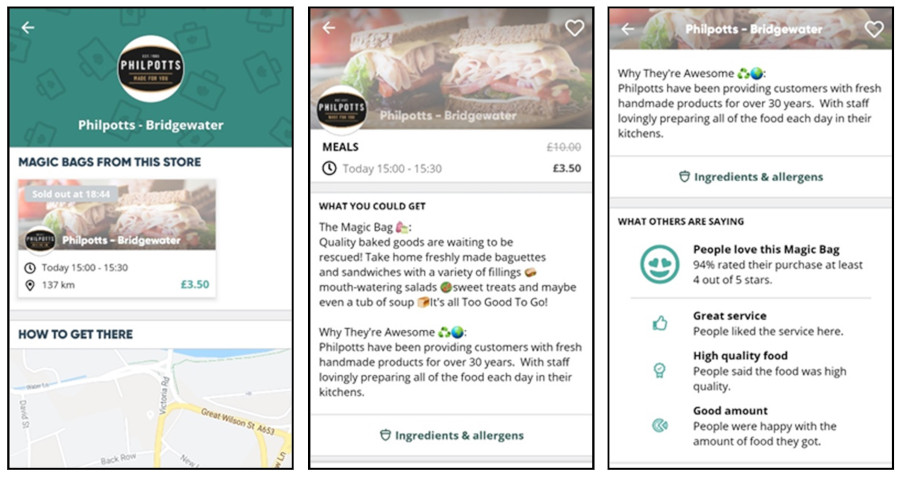The provided description details an image showcasing three separate screenshots of a place called "Fillpots" in Bridgewater as viewed on a mobile device. Here’s a refined and detailed caption based on the description:

---

### Caption:

**Overview of Fillpots in Bridgewater on Mobile Device:**

1. **Storefront Description:**
   The first image features the Fillpots logo in Bridgewater. The logo is set against a green background adorned with small suitcase icons that have heart shapes inside them. The central logo comprises a white circle with a black oval laid horizontally. The text "Fillpots" is displayed in bold white lettering.

2. **Magic Bags Sales Information:**
   Below the logo, bold capital letters announce the sale of "MAGIC BAGS" from Fillpots, which sold out at 18:44. The screen indicates a sales window earlier today, from 15:00 to 15:30, during which the magic bags were priced at £3.50. An embedded map shows the location of the store for easy navigation.

3. **Sandwich Display:**
   The final screen showcases a couple of sandwiches representative of the meals offered at Fillpots. Details reiterate the sale period for today's magic bags, echoing the price of £3.50. A comprehensive description follows, listing the contents originally included in the magic bag.

---

This refined caption provides a structured and detailed overview of the visuals, making it clear and informative for the reader.